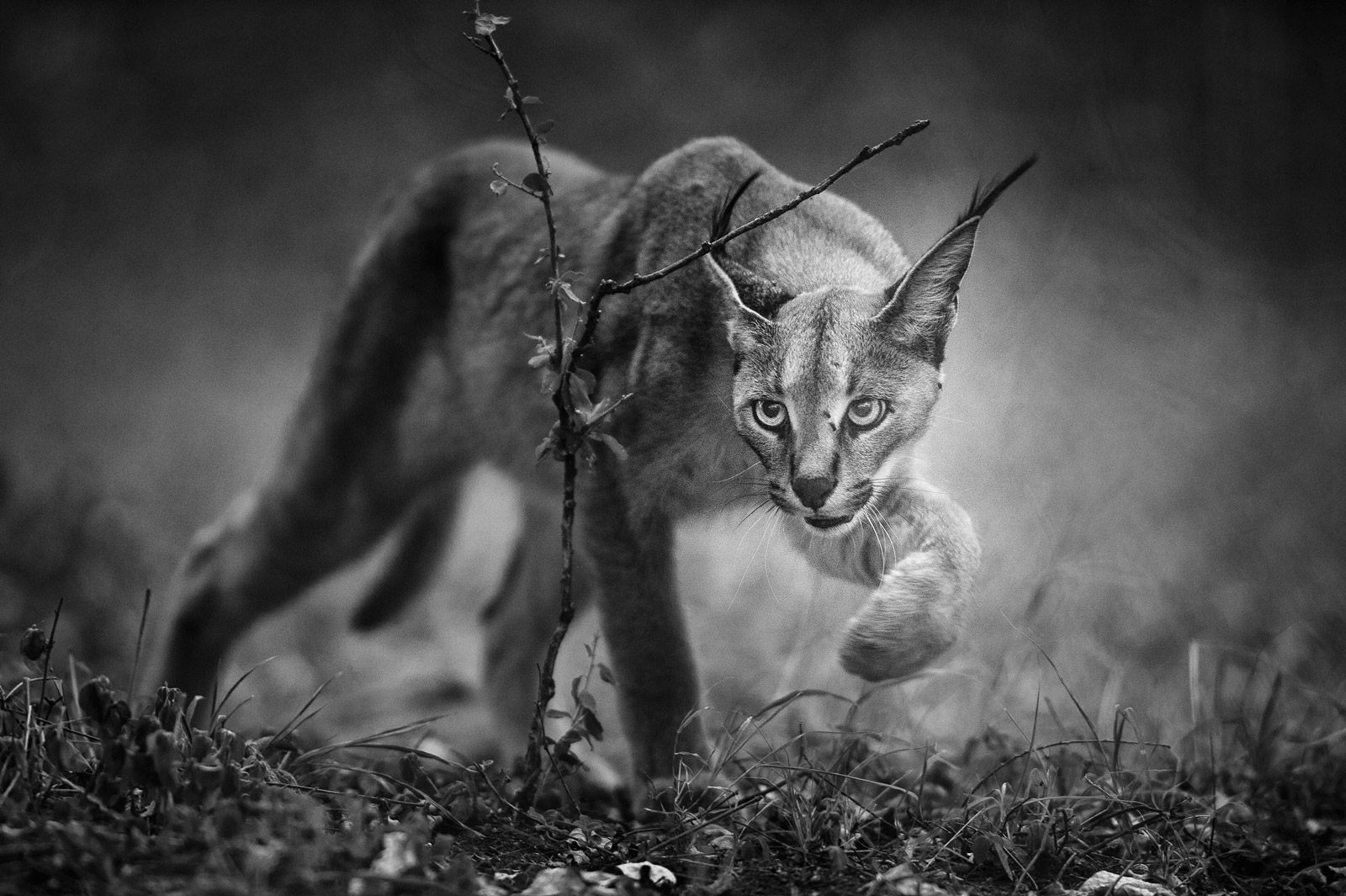This black and white photograph captures a large wild cat, possibly a lynx or similar type, walking directly towards the viewer through a grassy and leafy area. The cat's body extends off to the left side of the image, allowing a clear view of its size and muscular build. It has its front right paw on the ground while the left paw is lifted mid-step, indicating movement. A twig stands upright in the center foreground, adding a sense of scale and environment.

The cat's face, pointed directly at the viewer, is framed by tall, perky ears with noticeable tufts of fur at the tips, giving it an alert and focused appearance. The eyes are wide open with dark pupils, exuding a sense of determination likely as it stalks prey. White whiskers protrude prominently on both sides of its narrow, elongated snout. The fur exhibits various shades of darkness and lightness, from the crown of the head down to the tip of the nose, creating a striking contrast.

The background is blurred, consisting of a mix of grays, whites, and blacks, almost resembling an aura of smoke or fog, which adds a mysterious and ethereal atmosphere to the photograph. The monochromatic palette highlights the texture and intensity of the cat's fur and expression, making it the unmistakable focal point of the image.